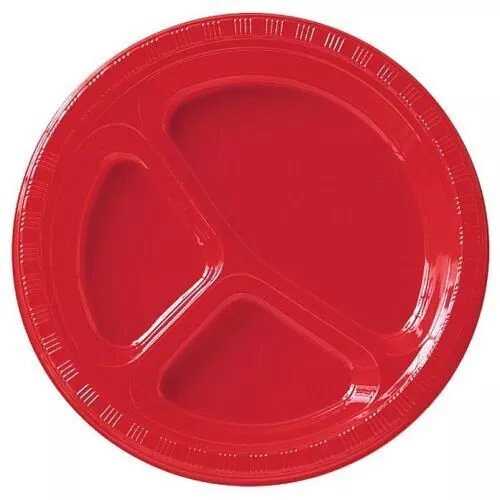This image depicts a stock photo of a shiny, red plastic disposable plate set against a white background. The plate, typically used for outdoor barbecues, church dinners, and birthday parties, features three compartments designed for food separation. The largest compartment, positioned at the bottom of the plate (or top right-hand corner depending on perspective), is ideal for main courses such as meats or bread. Two smaller, eye-shaped sections occupy the other side, perfect for side items like vegetables or fruits. The plate boasts a sturdy, simplistic design with a thick rim adorned by a subtle circular pattern of three lines interspersed with spaces, which continues uninterrupted around the edge. The plate’s reflective surface underscores its plastic material, making it a practical choice for casual dining and picnics.